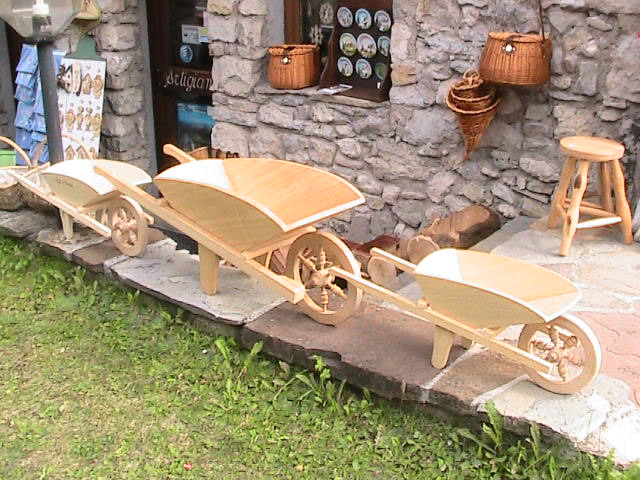The photograph captures an outdoor scene featuring a quaint stone building constructed from a variety of irregularly shaped rocks in shades of gray, pinkish-gray, light brown, tan, and dark gray, all fitted together. The building's facade includes a square wooden-framed window adorned with multiple round pictures or stickers, and nearby are a couple of woven wicker baskets, one placed on the ground and another hanging on the wall, including a unique funnel-shaped basket with smaller ones inside it. 

A chocolate brown door, embellished with numerous signs and pieces leaning against it, stands out on the building. Flanking the doorway are a couple of posters, adding a touch of character to the entrance, and a small, light wooden stool rests on the cobblestone pathway leading up to the door.

The cobblestone path itself is a medley of light gray, brown, and tan stones, bordered by light brown logs from a tree and leading down concrete steps. Alongside the path, three decorative wooden wheelbarrows of varying sizes—a small one, a large one, and a medium one—are lined up. The scene is set against a backdrop of light green grass, with a worn area in the left corner exposing light brown soil, creating a charming rustic aesthetic.